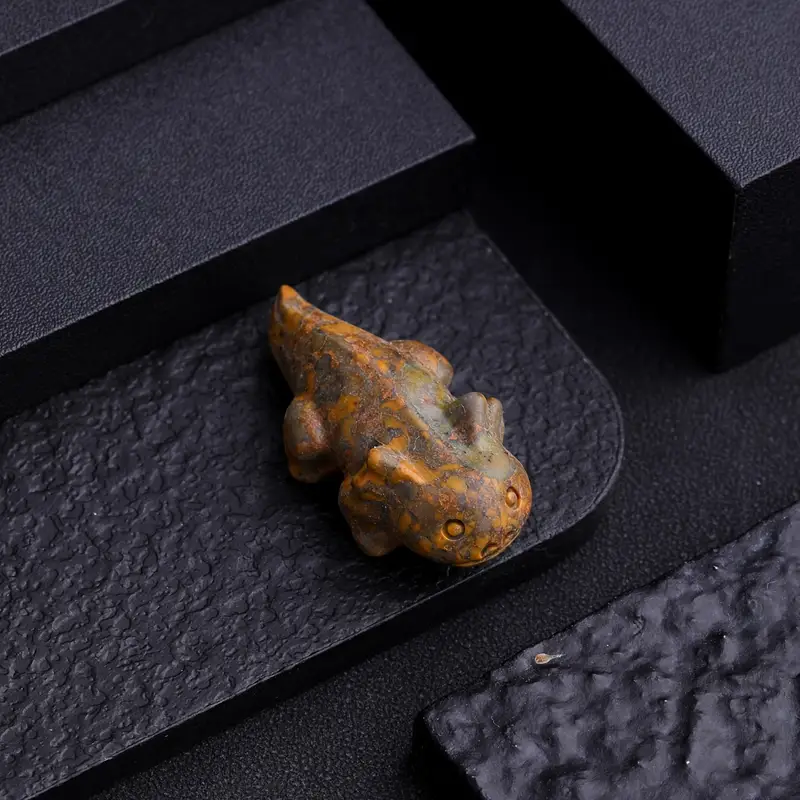The image features a detailed and colorful stone sculpture of an orange, amphibious-like creature—possibly a lizard or frog—situated prominently on a set of textured, black stone steps. The creature's design includes distinct features such as eyes, legs, tail, and a mouth, contributing to its lifelike appearance despite being a work of art. The creature, primarily orange with hints of brown and some green elements, rests on the bottom step in front of the viewer. The steps, which are rough and patchy in texture, lead in various directions, creating a dynamic background. The dominant colors in the image are black, orange, and brown, and there is no visible text, emphasizing the sculptural elements and the overall artistic composition.